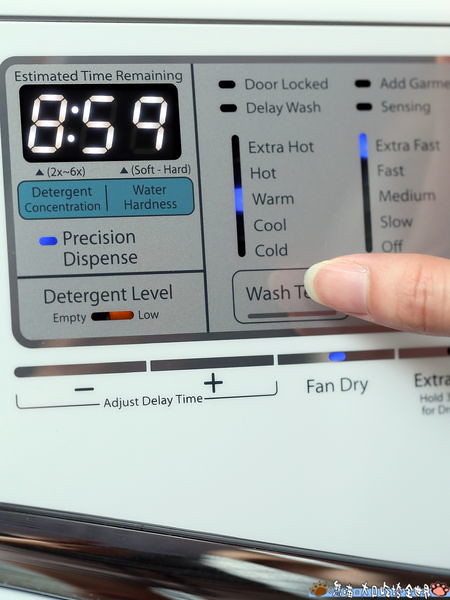In the image, a woman's thumb, characterized by a longer fingernail and appearing to belong to a white woman, is poised to press a partially obscured button labeled "wash something" on a high-tech washing machine's touch screen interface. The interface displays an estimated time remaining of 8 minutes and 59 seconds. The precision dispense light is illuminated, indicating attention to detergent levels, which are shown as low. Various other indicators such as door lock, delay wash, add garment, and sensing are present but not currently lit. The washing machine's water temperature is set to warm, which is highlighted in a blue light, and the spin speed is set to extra fast. The touch screen also features options to adjust delay time with plus and minus buttons and is part of a sleek design with a white exterior and a gray interactive panel.